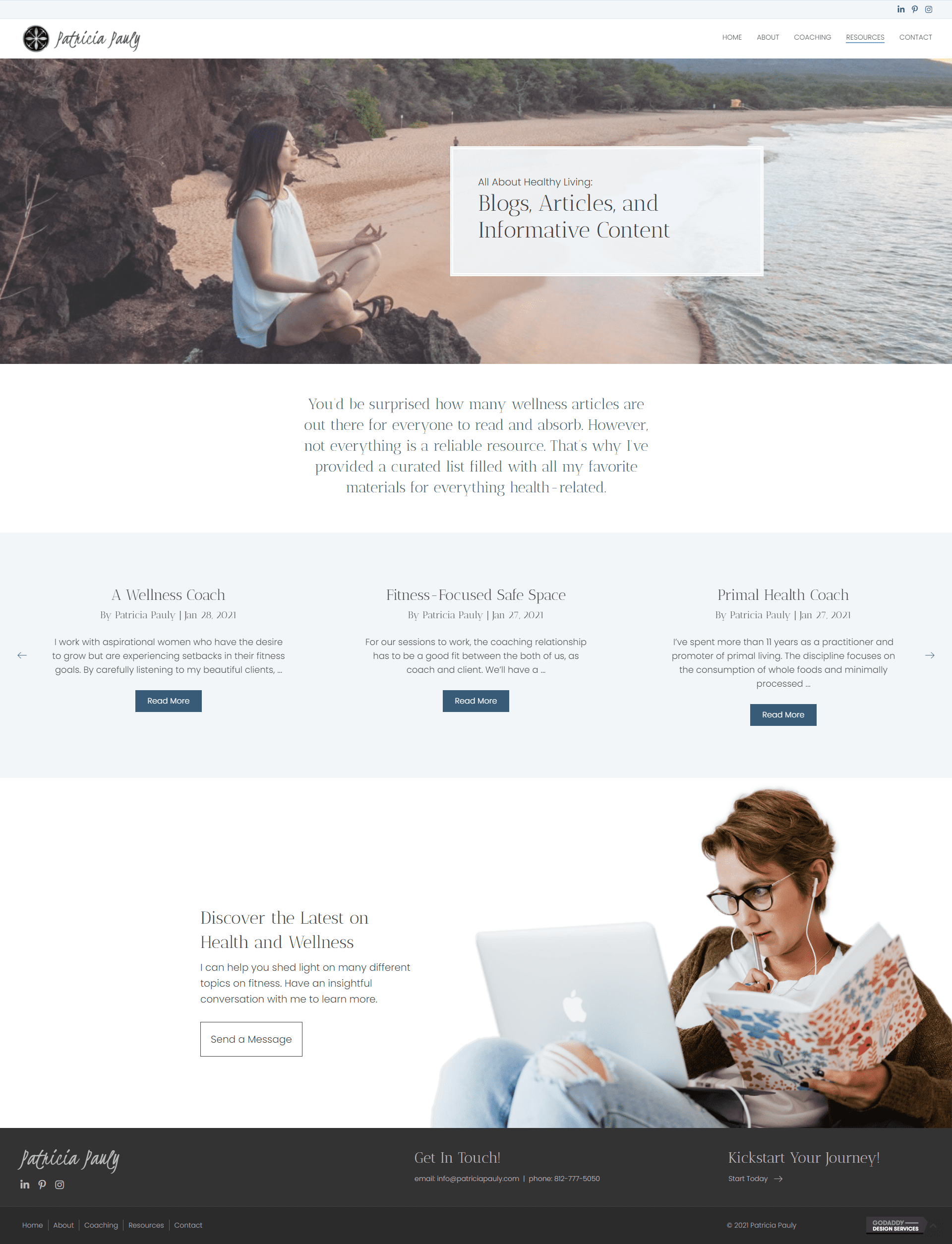Here is a cleaned-up and more detailed caption for the image:

---

The image showcases a website, potentially named "Patricia Pauly" with initials that might be FPA or MLY, although the cursive font and poor resolution make it difficult to discern clearly. This name appears in the top-left corner of the page. On the right side, there is a navigation menu with links labeled: Home, About, Coaching, Resources, and Contact.

Central to the page is a photograph of a woman, likely Patricia Pauly, sitting cross-legged with her hands in the "Ohm" position resting on her knees. She is wearing a white shirt, black shorts, and sandals, with shoulder-length hair.

A white rectangle on the page contains the text "All About Healthy Living - Blogs, Articles, Informative Content." Below it, another section on a white background reads: "You'd be surprised how many wellness articles are out there for everyone to read and absorb. However, not everything is a reliable source. That's why I've provided a curated list filled with all my favorite materials for everything health-related."

Underneath this text are three article titles, along with publication dates and "Read More" links in a teal color:
1. "Wellness Coach" by Patricia Pauly, January 28, 2021.
2. "Fitness Focus Safe Space" by Patricia Pauly, January 27, 2021.
3. "Primal Health Coach" by Patricia Pauly, January 27, 2021.

---

This detailed caption provides a clearer and more structured description of the website's elements and content.